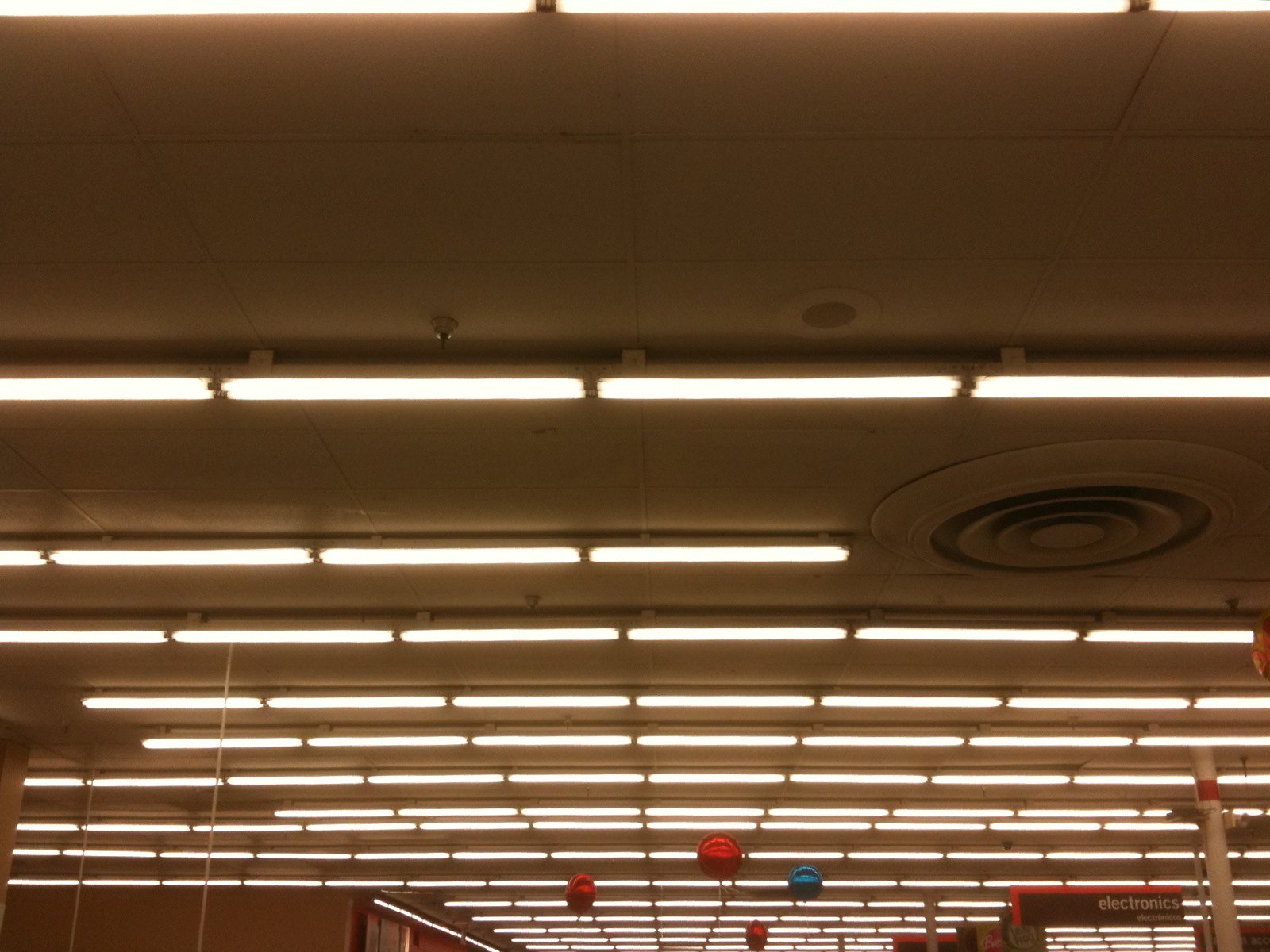The image depicts the interior of a store illuminated by rows upon rows of horizontally arranged fluorescent lights stretching across the ceiling. Visible on the ceiling are various fixtures, including fire sprinkler heads, a speaker, and an unspecified ventilation system. In the background, a clearly marked sign for the electronics section stands out, along with multiple other signs featuring a brown base color outlined in red. 

Adding a splash of color to the scene, clusters of red balloons have ascended near the ceiling, with at least one blue balloon visibly among them. On the right-hand side, there appears to be another balloon caught up high. A white pole with a red wrap near its top is also noticeable in the store. The walls are predominantly brown, and there are additional elements dangling from the ceiling by chains, likely signs or posters, though their contents are obscured from this vantage point.